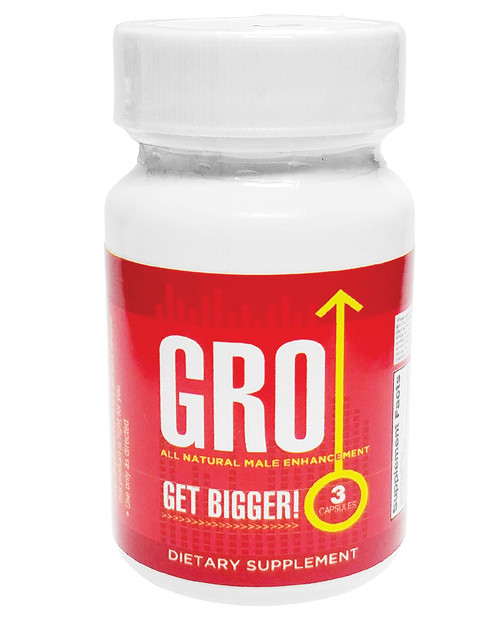This photograph features a white plastic medicine bottle, prominently positioned against a simple backdrop. The bottle has a distinct red stripe on the front, providing essential information about the product. The bold white letters on the red background spell "GRO," and just below it, in yellow, the label reads "ALL NATURAL MALE ENHANCEMENT." Further down, in white text, the label exclaims "Get Bigger!" A white number "3" is situated to the right, encapsulated within a yellow circle. An elongated arrow, also in white, points upwards, traversing past the "O" in "GRO." The overall image focuses closely on the bottle, giving prominence to its detailed labeling and branding.